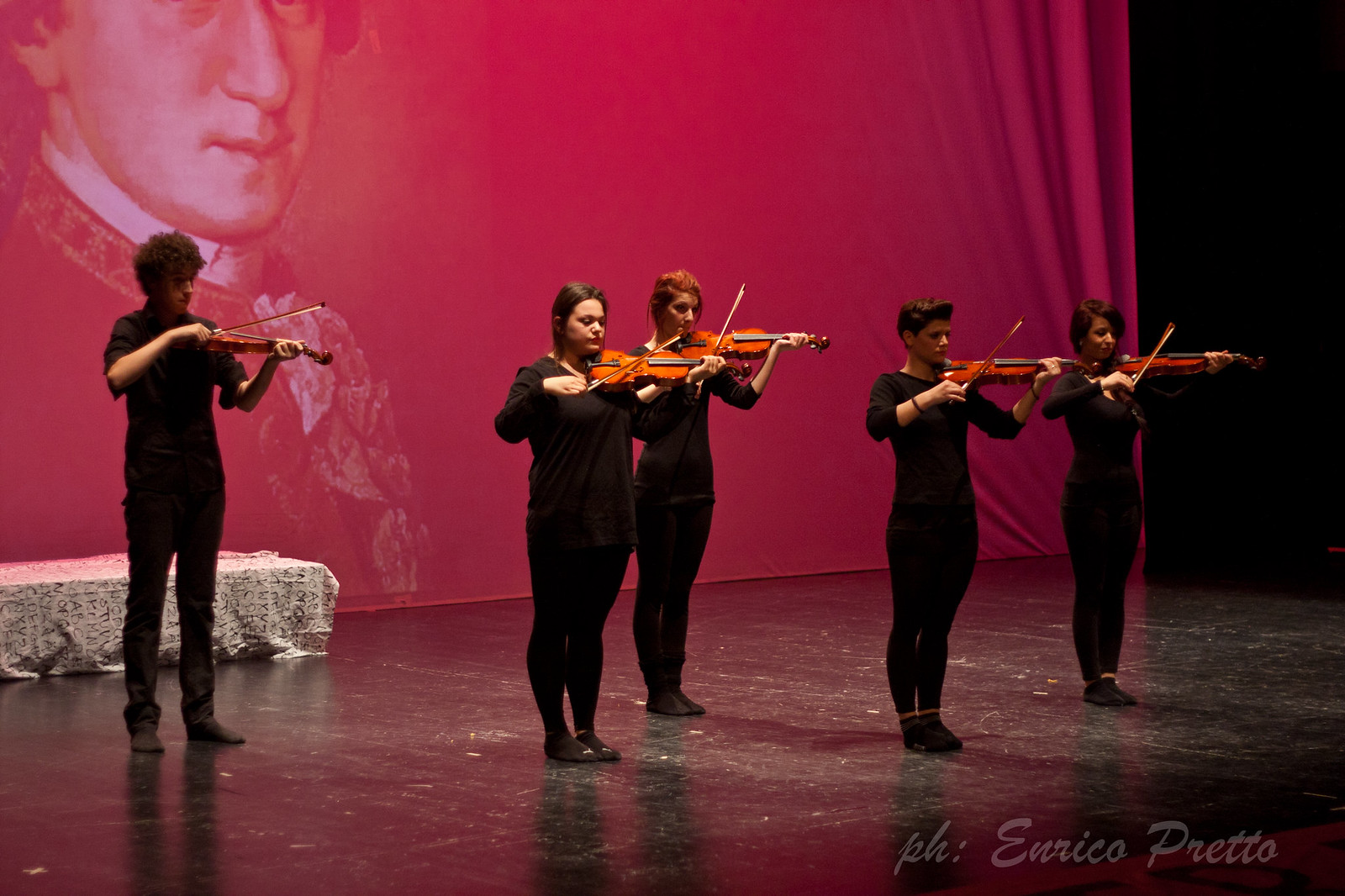In the photograph, five violinists are captured performing on a stage. The ensemble consists of three women and two men, all elegantly dressed in black long-sleeve tops, black pants, and dark shoes, with violins made of reddish wood. One notable female violinist stands out with her red hair among the predominantly dark-haired group. They exhibit excellent posture while playing, with one tall male violinist uniquely pushing the violin up against his shoulder rather than holding it with his chin.

The stage floor is black with chips revealing white underneath, adding to the photograph's texture. In the backdrop, a rich red curtain dominates with a partially visible image of what appears to be a historical figure, possibly George Washington, dressed in fancy clothes with a frilly ascot. On the lower left side of the image, the photograph is credited to Enrico Preto, denoted by "ph colon." The setting includes a bench draped with white printed fabric, and the upper right corner of the backdrop sports a black section, providing contrast. Overall, this detailed scene captures a moment of musical performance and visual intricacy.